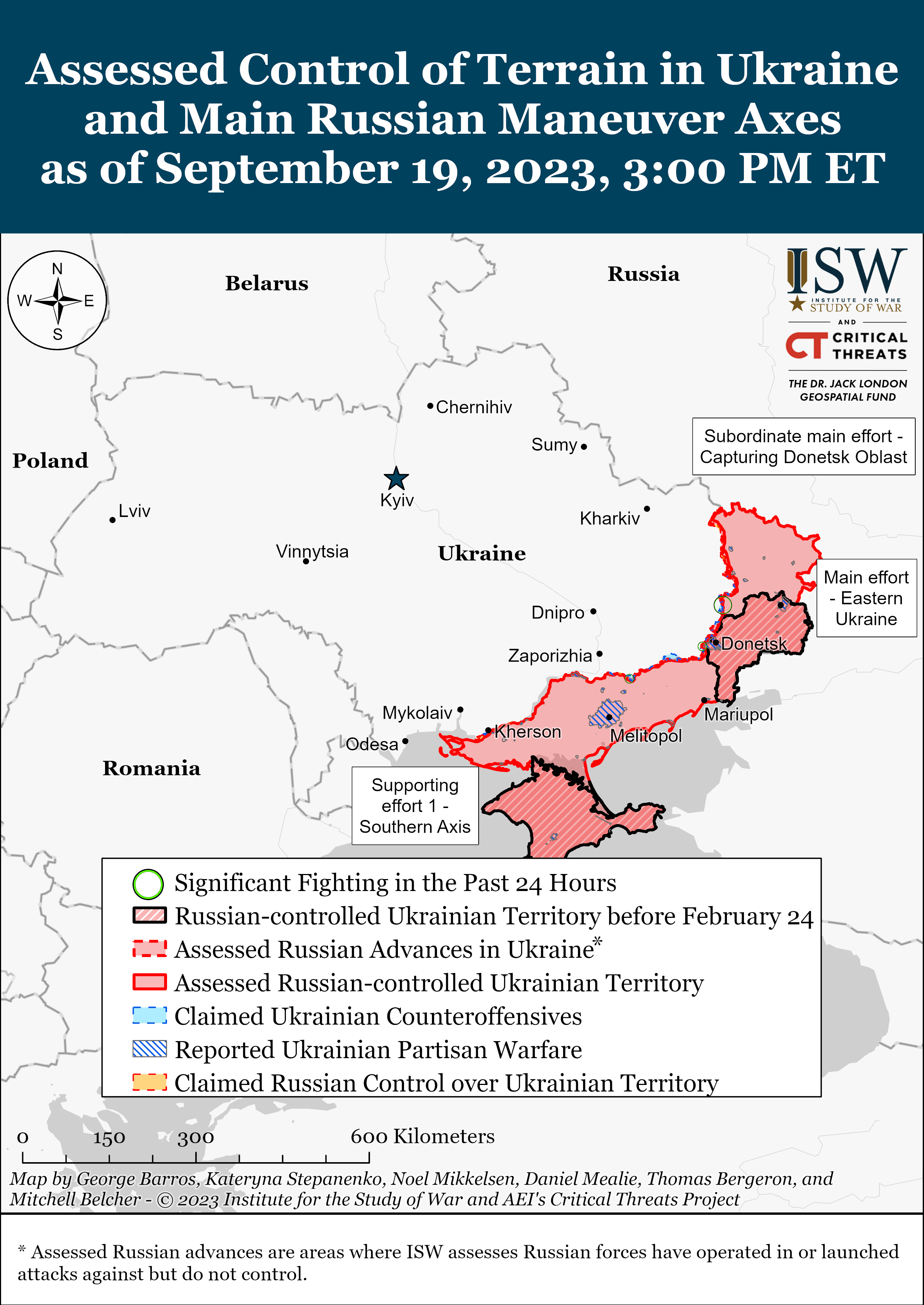This image is an informational publication showcasing a detailed map of Ukraine and adjacent countries like Russia, Romania, Poland, and Belarus as of September 19, 2023, 3:00 p.m. Eastern Time. The top of the map is marked with a dark blue banner inscribed with white text that reads, "Assessed Control of Terrain in Ukraine and Main Russian Maneuver Axes." This map primarily highlights the areas of eastern Ukraine under Russian control, depicted in various shades of pink and red, and includes a comprehensive legend that deciphers the different colors and shadings used to denote Russian-controlled territories, areas of significant fighting, reported Ukrainian partisan warfare, and claimed Ukrainian counteroffensives. Additionally, the map features scales to measure distances in kilometers, providing spatial context. In the lower section, there is a box explaining that "Assessed Russian Advances" are regions where the Institute for the Study of War (ISW) assesses Russian forces have operated or launched attacks but do not fully control. The publication also notes contributions from institutions like the Critical Threats Project and the Dr. Jack London Geospatial Fund.